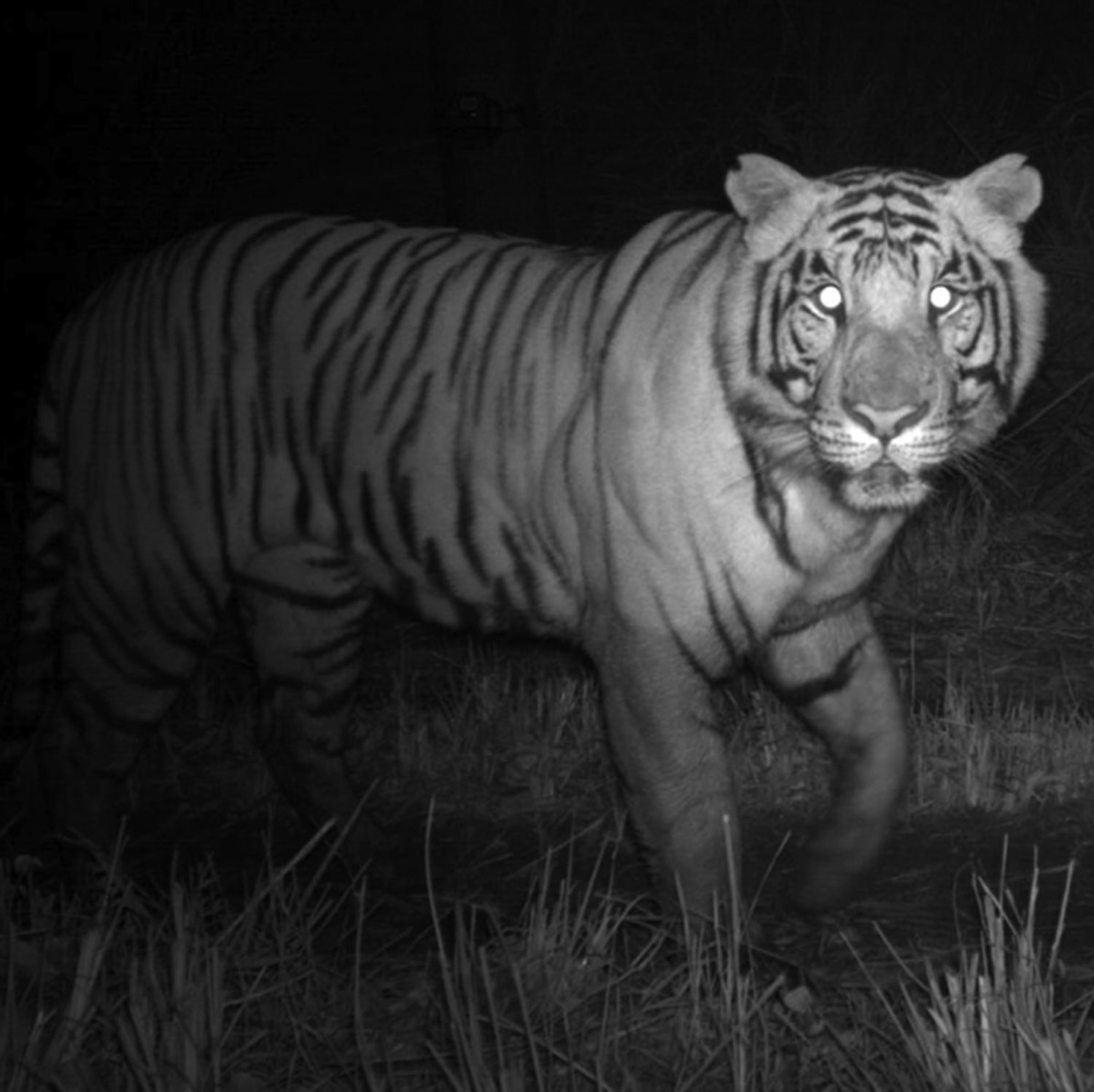The nighttime black-and-white photograph captures a majestic tiger standing still in an open grassy area, intensely staring directly at the camera with vivid, glowing eyes illuminated by a flash. His posture is striking, with his left paw lifted mid-stride, suggesting he was in motion before being momentarily frozen by the shot. The short grass allows a clear view of his entire body, highlighting the beautiful stripes that define his massive frame, including the distinctive patterns around his face and body. The upper portion of the image is primarily dark, creating a stark contrast with the visible weeds and the tiger's alert ears, emphasizing his natural habitat and possibly hinting at an instinctual hunt. The photograph’s lack of text and color enhances the raw beauty and wild essence of the scene.